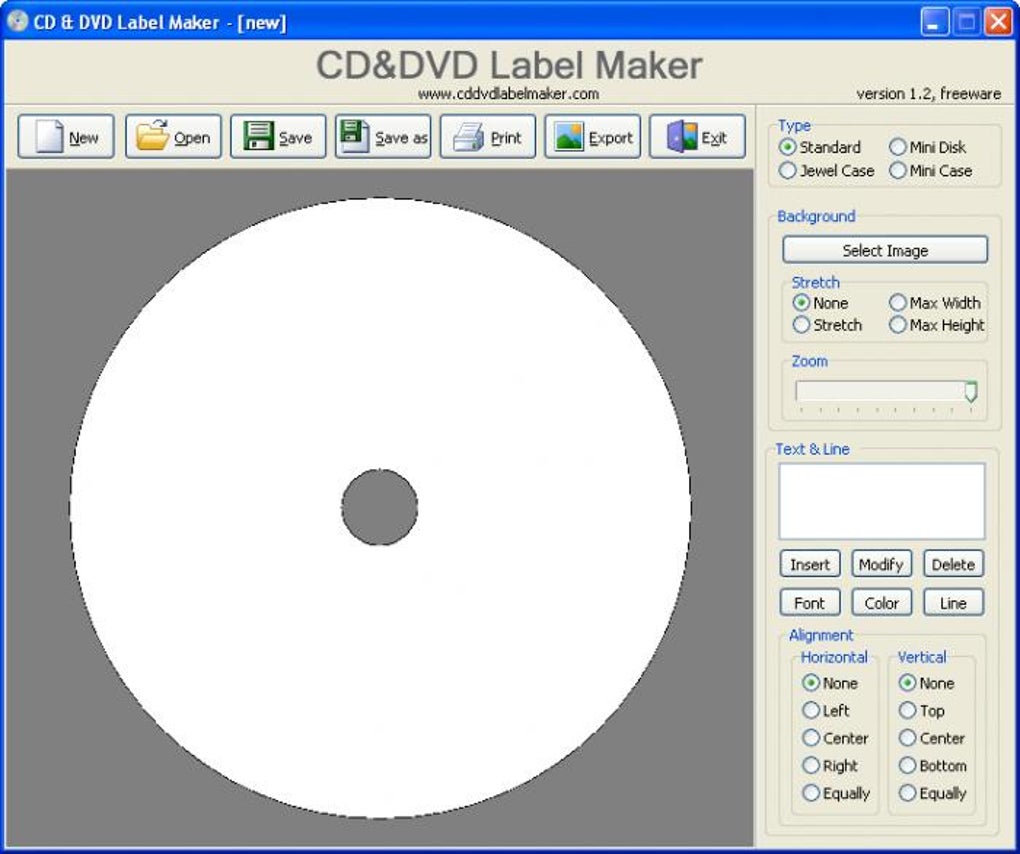The image is a screenshot of a computer program named CD and DVD LabelMaker, which appears in an older version of Windows with the familiar blue border. Prominently displayed at the top is the program name, "CD and DVD LabelMaker," along with the website URL and the text "Version 1.2 Freeware." In the upper right-hand corner, the standard minimize button and red X for closing the window are visible. The background of the software interface is a light gray.

At the top of the interface are classic icons typical of older Windows versions: "New," "Open," "Save," "Save As," "Print," "Export," and "Exit," each accompanied by corresponding icons, such as a file folder for "Open" and a floppy disk for "Save." The left side of the main area features a solid white CD image, which occupies a significant portion of the screen space.

On the right side, running vertically along the entire length of the interface, is a panel with various customization options. These options include selecting different types of discs or cases (Standard CD, Minidisc, Jewel Case, Minicase), changing the background (Select Image, Stretch, None, Max Width, Max Height, Zoom), and text modifications (Insert, Modify, Delete, Fonts, Color, Line, Alignment with horizontal and vertical settings).

The color scheme includes shades of beige, blue, yellow, orange, green, purple, red, white, gray, and black, giving it a nostalgic, early-2000s look.